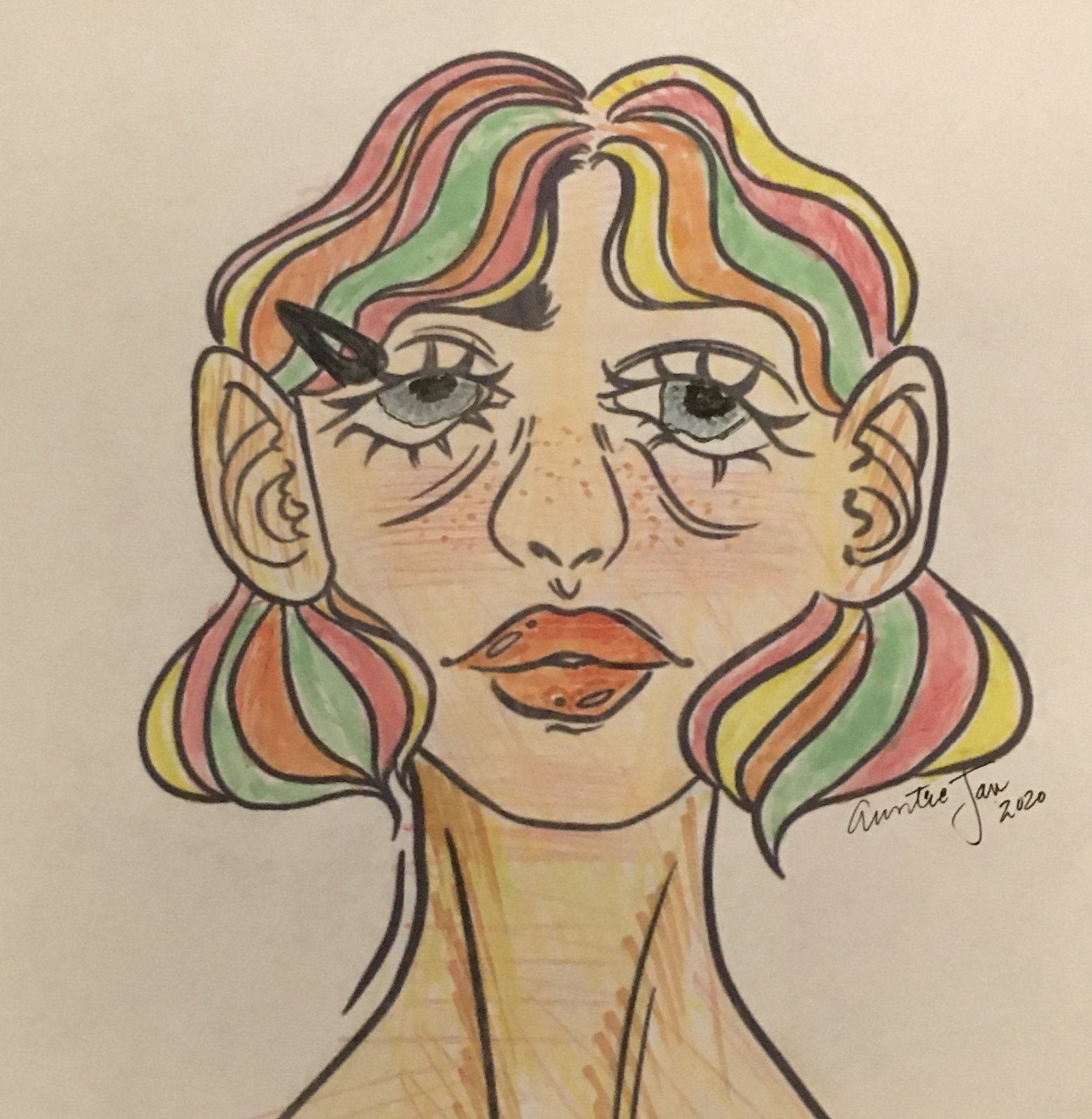The image is a caricature drawing of a Caucasian woman with a bob hairstyle, distinguished by its vibrant, rainbow-colored strands. Her hair features hues of pink, yellow, orange, and green arranged in a captivating rainbow pattern, falling just past her chin. This bob is accessorized with a hairpin positioned above her right eye, partially covering her face. The woman has striking blue eyes emphasized by long eyelashes, and her facial features include big red lips and a hint of blush on her cheeks, which contrast with her otherwise natural, makeup-free appearance. She also has subtle freckles around her nose, though they are faint and difficult to notice. Notably, only one eyebrow is visible in the drawing. Her slender neck adds to the caricature's characteristic exaggerated style. There is text beneath the drawing that reads "Jan 2020," along with a name that seems to be either "Amy" or "Ain," likely referring to the artist or the subject of the caricature.